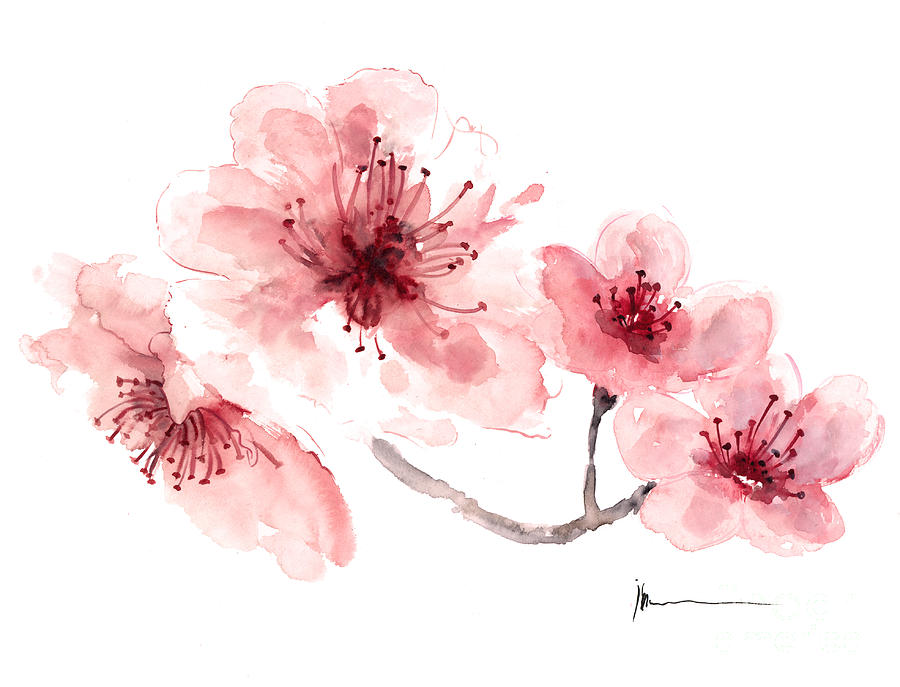This image depicts a detailed painting of four pink flowers in full bloom, attached to a gray, slightly squiggly branch. The flowers, which are not real but artistically rendered, each exhibit five to eight petals that transition from almost white at the edges to deeper pinks and reds toward the center. The central parts of the flowers showcase dark red filaments or stamens, with distinct circular tips. Positioned in various parts of the image, one large flower faces downward on the bottom left, another prominent bloom rests towards the top right, while the remaining two flowers are located near the bottom right and upper left. The branch connecting these flowers traverses the painting, starting from the middle, moving downwards, and then curling up towards the bottom right. A signature, featuring what appears to be the initials "JH" followed by a scribble, is located in the bottom right corner.